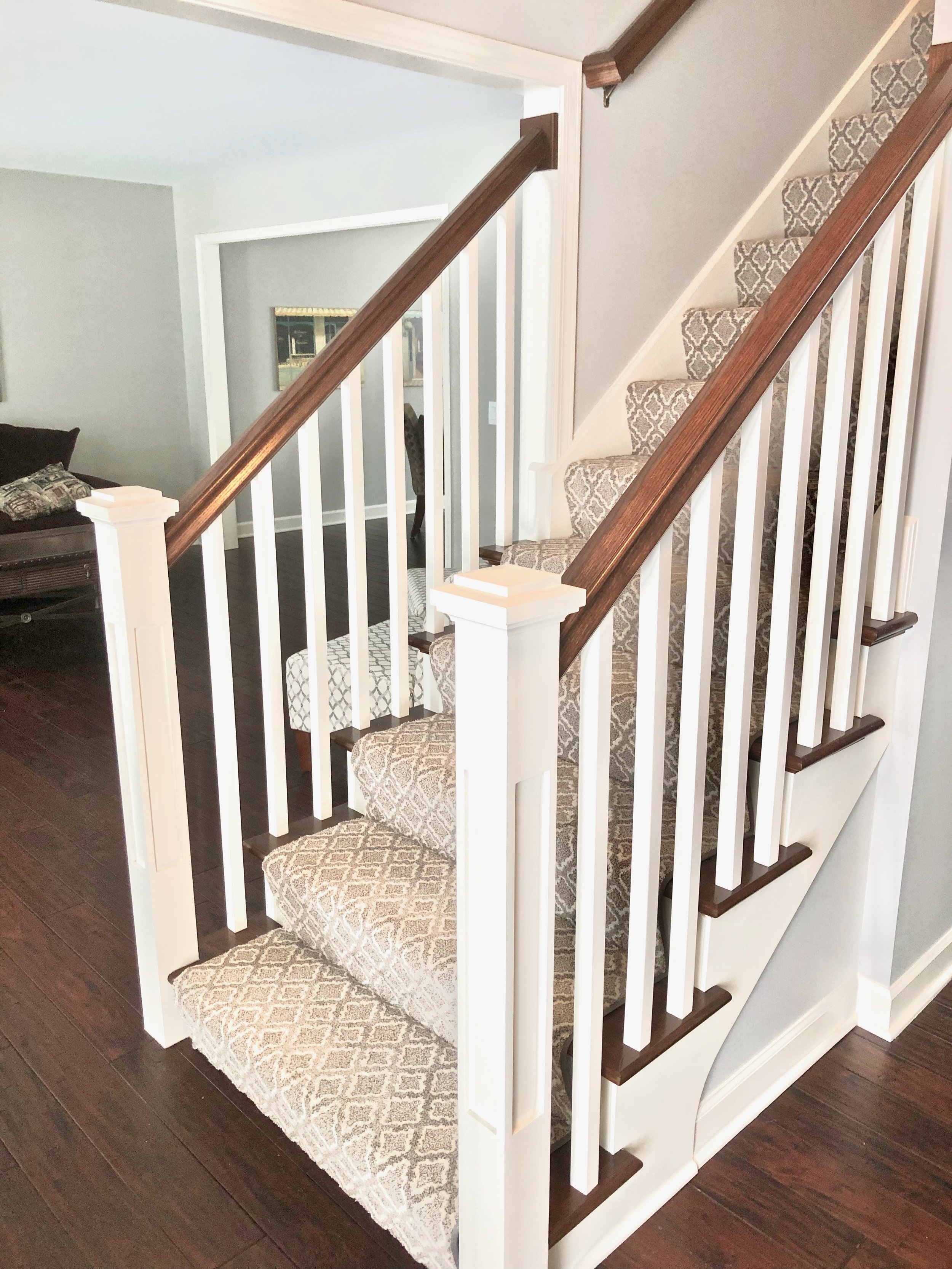This image captures the interior of a house, primarily featuring a staircase that ascends from the bottom left to the top right. The staircase is straight with polished wooden handrails reflecting warm yellow light, enhancing its natural walnut hue. The stairs are covered with a gray and beige carpet, adding texture. In the middle right of the image, there's a beige-gray couch positioned near an open doorway base, revealing an adjoining room, possibly the dining area. The first floor showcases dark wooden flooring, polished to reveal intricate textures. Additional subtle details include white frames or columns around the staircase and a hint of a mirror and possibly a wooden chair in the background. The setting appears somewhat sparse, giving an impression of openness and space.